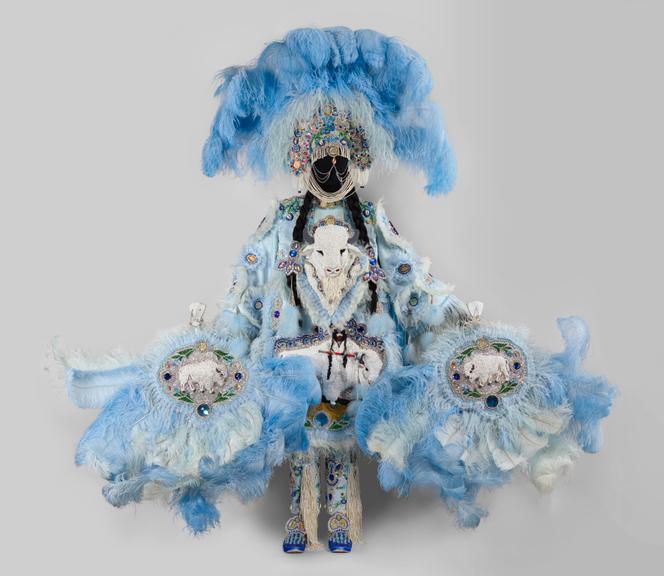The image features an elaborate faceless doll or mannequin adorned in an ornately designed costume. The centerpiece of the outfit is a striking headdress made of large, vibrant blue feathers that tilt slightly downwards, interspersed with multiple colors including oranges, yellows, pinks, and purples. The costume extends down to a broad, dress-like bottom, predominantly in blue and white hues, embellished with an array of feathers and glittering gems. The chest of the figure features a pure white image of a lamb or cow, facing forward. Furthermore, the doll wears a black mask, adding to its mysterious appearance, and the arms display rows of downward-facing feathers encircling the wrists. Two medallions or emblems are embedded on the sides, adding to the costume's opulence. The outfit also includes similarly designed blue shoes and pants, completing the striking ensemble.